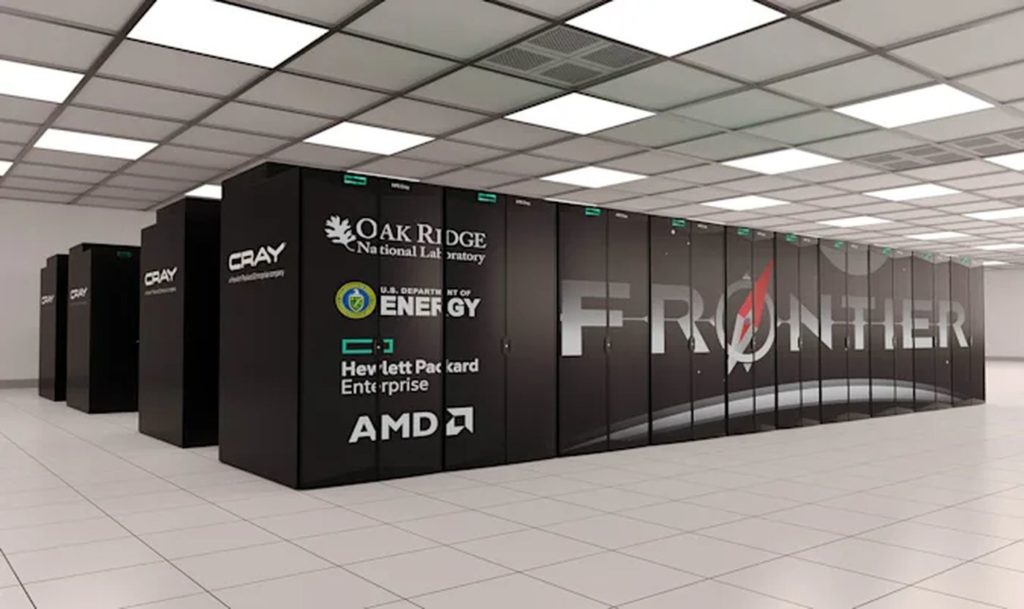This image depicts the interior of a large room featuring a tiled floor and a drop ceiling composed of large white and gray panels, some of which are illuminated with fluorescent lighting. Inside the room are four rows of tall, vertical locker-like units, presumably housing a supercomputer. The forefront row prominently displays the word "Frontier" in large, capital gray letters with a distinctive red and white directional symbol over the "O". Below the main row, the leftmost unit bears several labels in white text: "Oak Ridge National Laboratory" with an adjacent leaf icon, "U.S. Department of Energy" accompanied by a green and blue symbol, "Hewlett Packard Enterprise" alongside a small blue box, and "AMD" marked with an upward-diagonal arrow. On the side, "Cray" is printed in white letters with additional smaller text beneath it. The entire setup, spanning four rows from front to back, is situated centrally in the room, suggesting it serves as a major computing resource, likely for official or research purposes. The overall color scheme features shades of gray, white, black, turquoise, and red, accentuating the high-tech and institutional ambiance of the space.